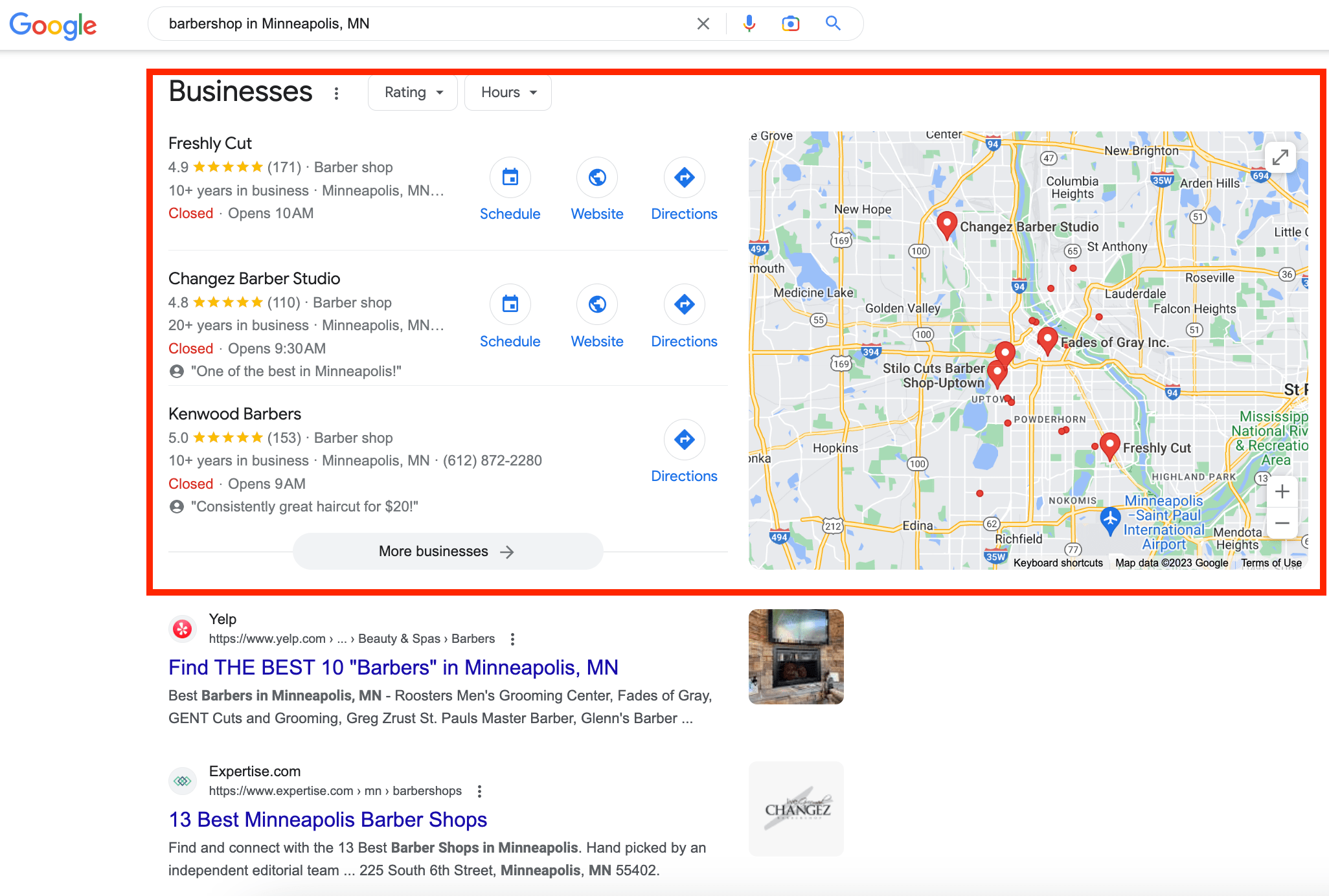The image is a screenshot of a Google search for "Barbershop in Minneapolis, MN." The Google logo is visible in the top left corner. In the search results, several barbershops are listed, including "Freshly Cut," "Changes Barber Studio," and "Kenwood Barbers," highlighted by a red rectangle. Beside these listings is a map on the right, dotted with red pinpoints indicating various barbershop locations in the area. Below the business listings, additional search results appear. The top link is from Yelp, titled "Find the Best 10 Barbers in Minneapolis," accompanied by a thumbnail image of a barbershop interior. The second link is from expertise.com, titled "13 Best Minneapolis Barbershops," featuring a thumbnail with the Changes Barbershop logo.